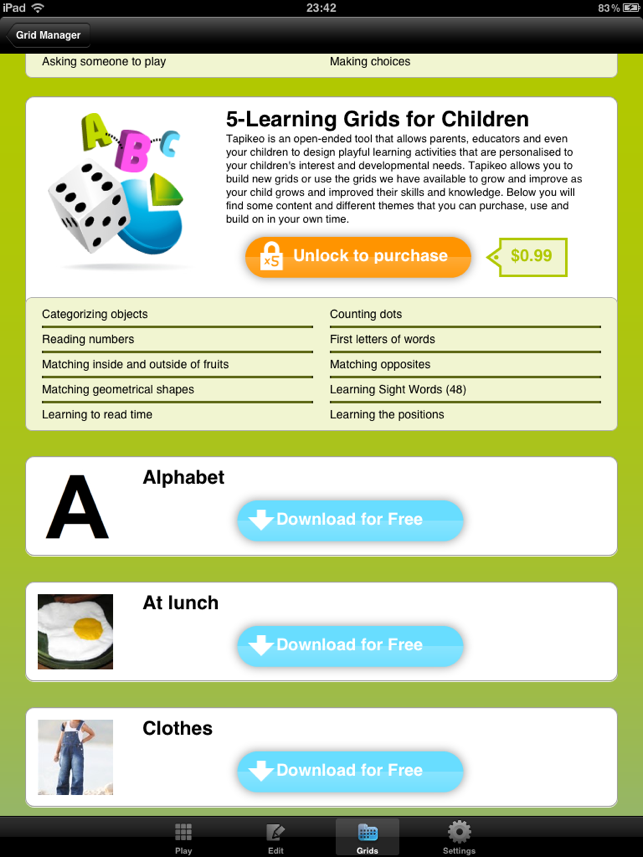The image displays an iPad screen featuring a website interface specifically designed for setting up educational tools for children. At the very top of the screen, the iPad status bar is visible, showcasing standard information such as the battery level and other status icons, confirming the device in use. The central focus of the webpage is on a "Grid Manager" specifically targeted toward managing learning grids for children. Prominently advertised in the middle of the screen is an option to unlock additional features for $0.99, indicating a purchase mechanism embedded within the app. Surrounding the description of the learning grid are small, animated illustrations including a dice, a pie chart, and colorful, interconnected letters, adding a playful and educational visual appeal. Below these visuals, a detailed listing describes various accessible features within the learning grid, aimed at assisting parents in enhancing their children's educational experiences.